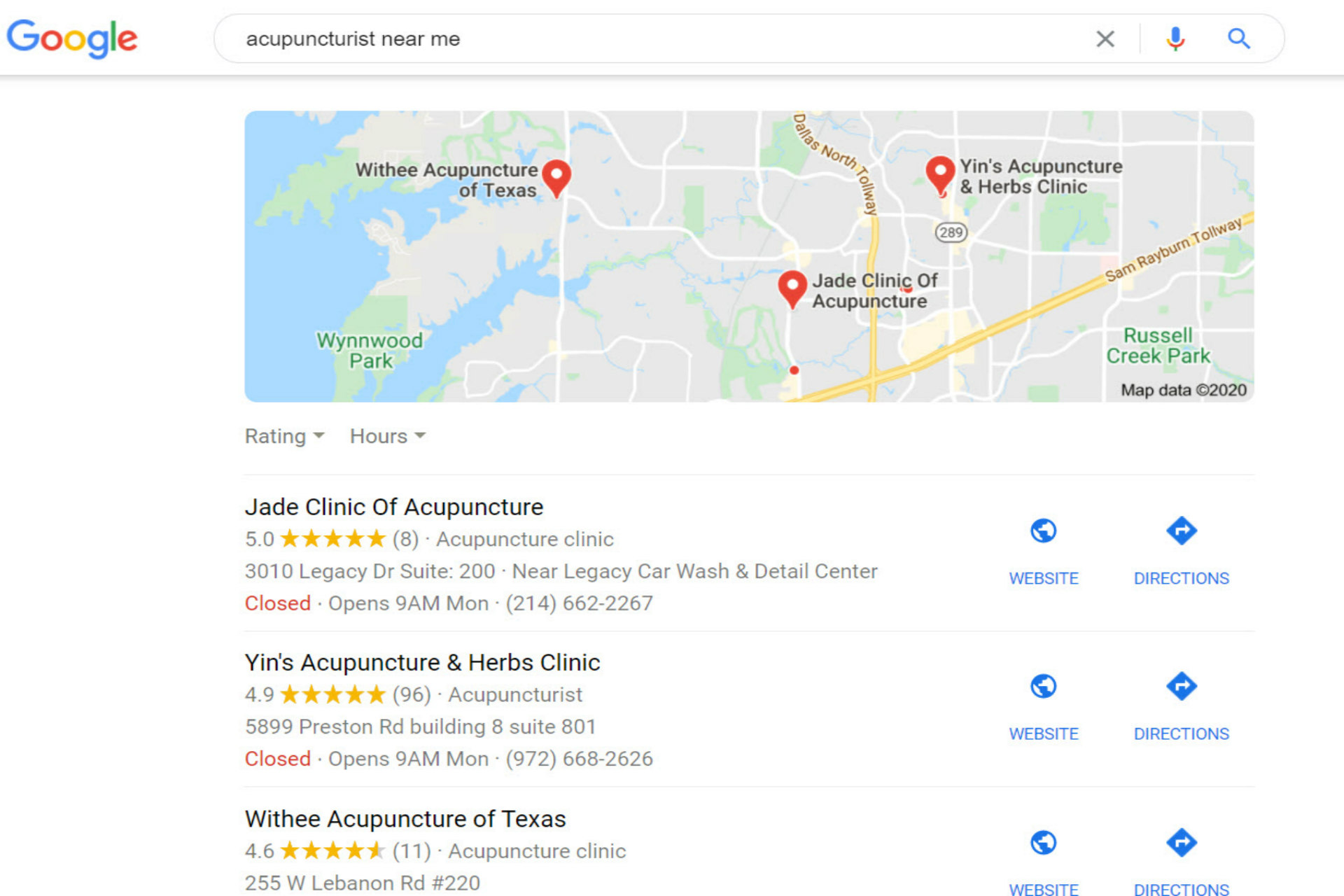The image depicts a detailed Google search results page for the query "acupuncturist near me." 

In the upper left corner, the recognizable Google logo is displayed. Adjacent to it, the search input field contains the text "acupuncturist near me." At the far right of the search bar are various icons: an 'X' for clearing the input, a microphone icon for voice searches, and a magnifying glass symbol to initiate the search.

Beneath the search bar, a map showcases three highlighted locations of acupuncturists. Below the map, on the left, are drop-down options for "Rating" and "Hours." The search results are presented in a structured list format underneath this section.

The first result is for the Jade Clinic of Acupuncture. The clinic’s name is displayed in bold black font, followed by a gray font indicating it has a five-star rating from eight reviews. The address is listed, and the status "Closed" is shown in red, signifying the clinic's current status. The star ratings are highlighted in yellow.

Similarly formatted, the second result is for the "Acupuncture and Herbs Clinic," and the third result is for the "Acupuncture of Texas." To the right of each listing are icons: a blue globe symbol representing the website, and a directions icon for navigating to the location.